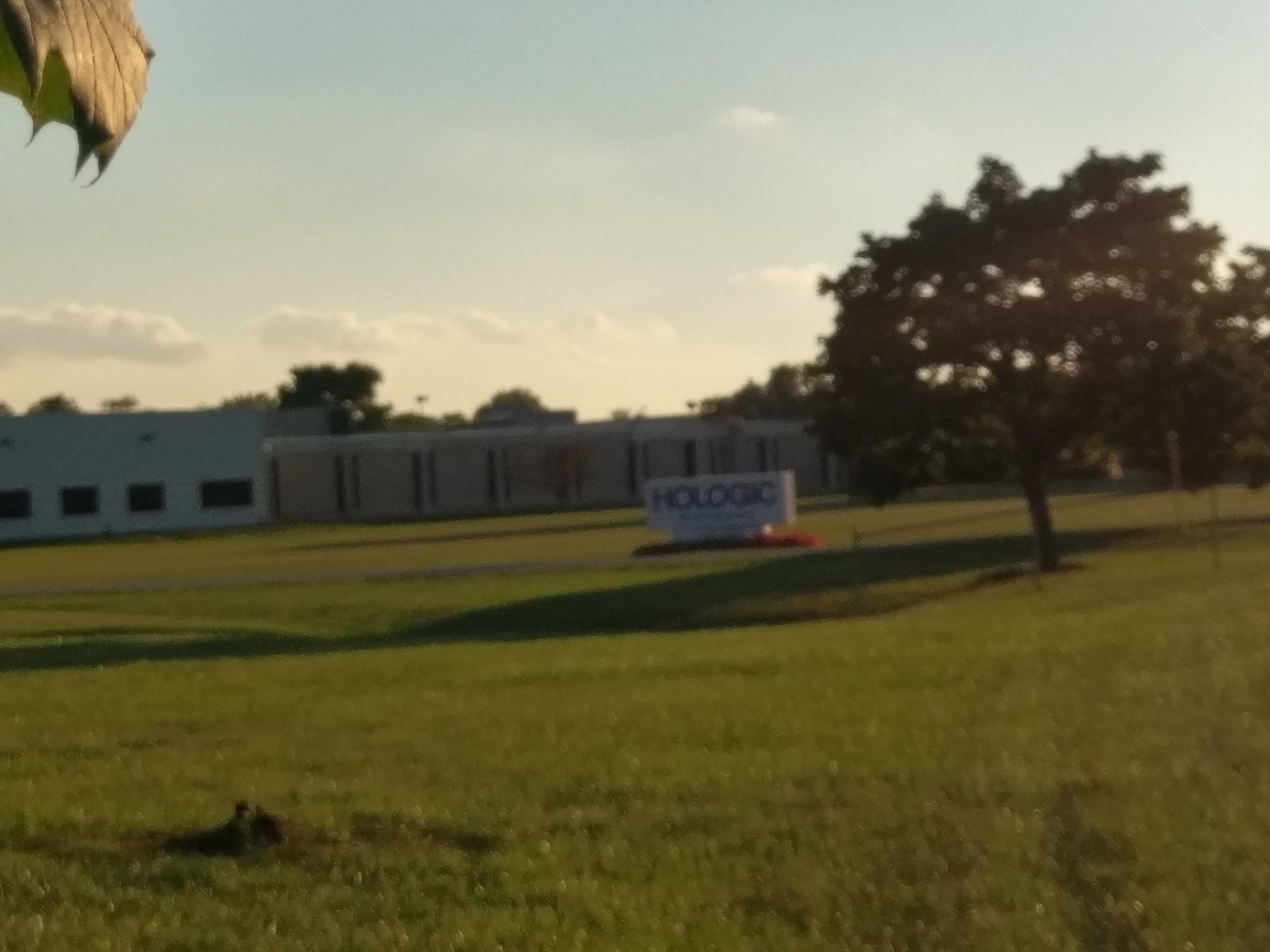A serene grassy field forms the foreground of the image, stretching towards the horizon. In the distance, there stands a white stone sign embedded within a reddish patch of ground. The sign bears the inscription “HALOGIC” in bold, capital letters. To the right of the sign is a large, vibrant green tree, with additional trees dispersed throughout the background.

On the left side of the field, slightly behind the sign, two distinct buildings are visible. The first is a gray building adorned with narrow black lines resembling windows. Adjacent to it on the left is a larger white building featuring dark, rectangular windows that create a contrasting visual pattern.

The sky above transitions from a deep blue at the top to a lighter hue near the bottom, where a few clouds drift lazily. In the top left corner, a lone leaf catches the sunlight, reflecting a bright glint. Meanwhile, a curious hole punctuates the ground in the bottom left of the image, adding an element of intrigue to the tranquil scene.